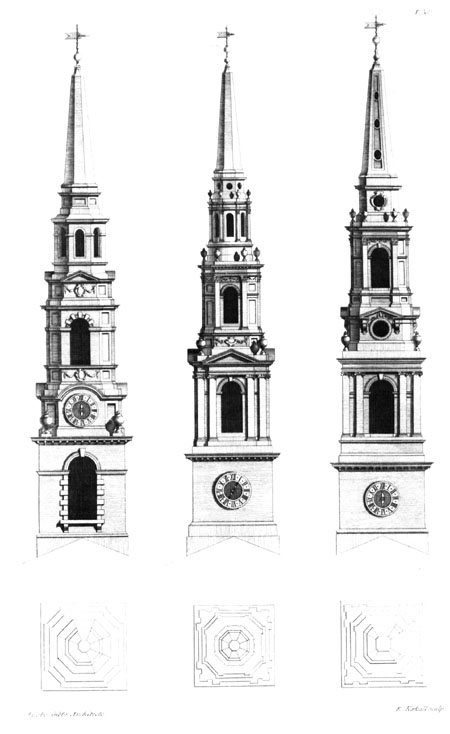The image presents a detailed illustration of three black and white, cathedral-like buildings, each with a distinctive pointed steeple adorned with a cross at the top. The structures feature prominently triangular rooftops and dark black windows that contrast with the light gray sides and tops of the buildings. The architectural designs, although similar in their Gothic style, vary subtly from one building to the next, each showcasing different arrangements and numbers of arches and window placements. At the bottom of the image, smaller segments appear to represent additional details or patterns, possibly instructional fragments that suggest a progression in the complexity of the building designs. This creates an impression of an instructional guide on the evolution of architectural styles from one building to the next.